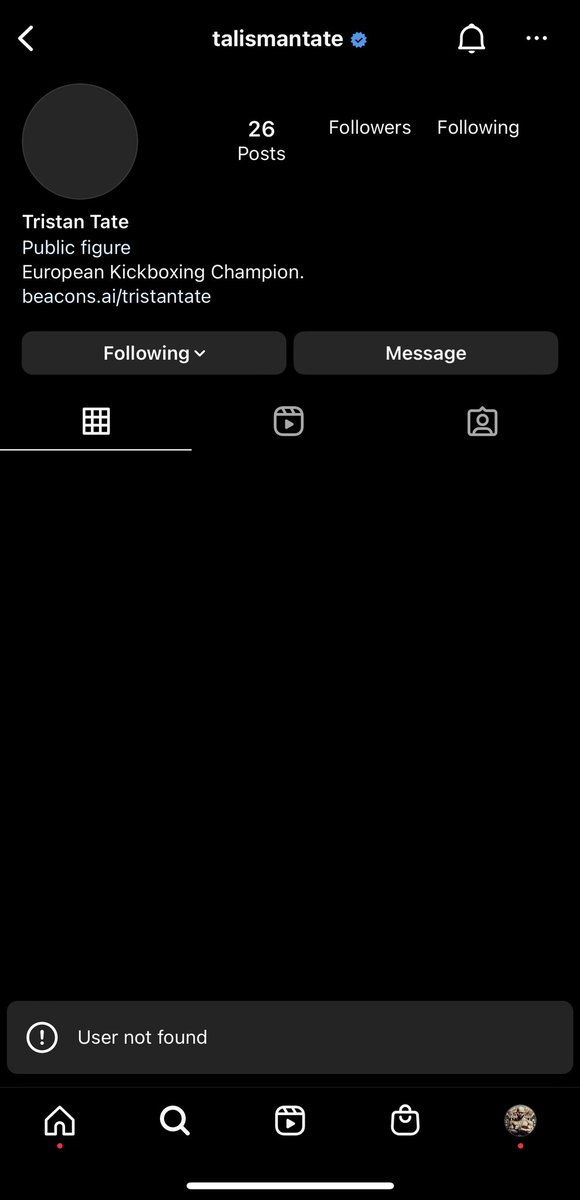A detailed screenshot of a Twitter profile page:

The screenshot captures a Twitter profile page in a dark mode theme with a black background and white text. 
- **Top Section**: At the top left, a left-arrow icon indicates a back navigation option. Centrally, the username "Talisman Tate" is displayed with a blue checkmark next to it, signifying a verified account. Adjacent to the username are a white bell icon (for notifications) and a three-dot menu icon.
  
- **Profile Area**:
  - The username is clarified as "Tristan Tate".
  - There is no avatar image; instead, a gray circle indicates the absence of a profile picture.
  - Beneath this, it reads: "Tristan Tate, public figure, European kickboxing champion, beacons.ai/TristanTate."
  - The profile information indicates "26 posts" without displaying the number of followers or following accounts.
  
- **Action Buttons**: Below the profile information are two gray buttons:
  - One button labeled "Following" in white text.
  - Another button labeled "Message" in white text, located to the right of the first button.
  
- **Profile Navigation**: Below the action buttons, there are three icons in white text:
  - A grid icon (highlighted, indicating the current view),
  - A play button for videos,
  - A profile picture icon.
  
- **Bottom Notification**: A gray rectangle with an exclamation point inside a circle contains the message "User not found," indicating issues with the profile's visibility or existence.
  
- **Footer Icons**: At the very bottom, there are five icons aligned horizontally:
  - A home icon,
  - A search icon,
  - A video icon,
  - A shopping bag icon,
  - A user profile icon (depicting a person with folded arms and a red dot beneath it).
  
- **General Layout**: The entire interface maintains a monochromatic theme, with a dominant black background and white text elements, creating a stark contrast for readability.